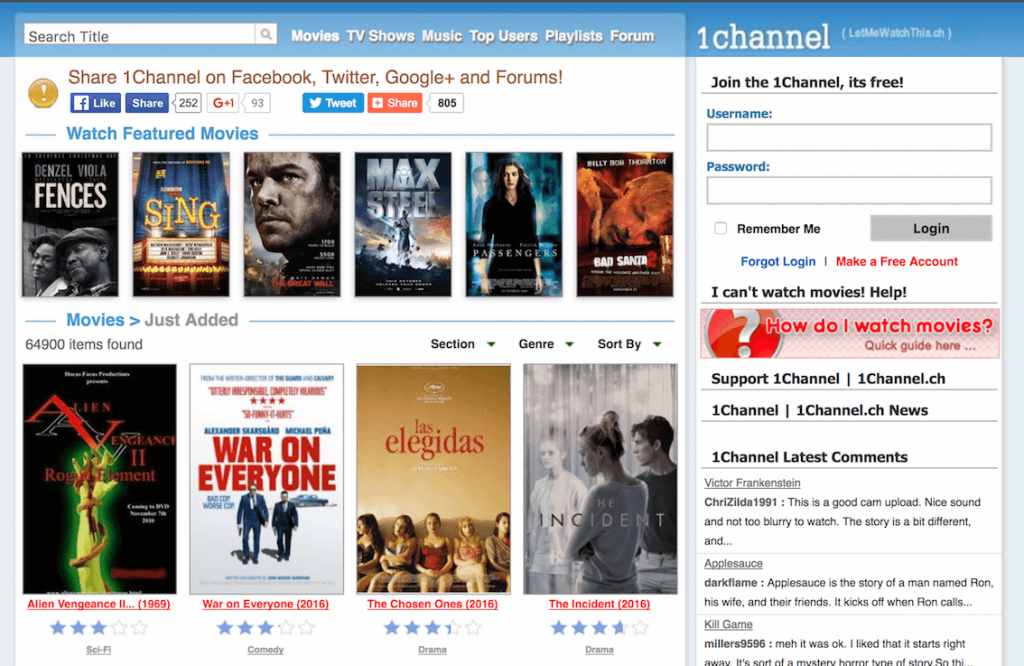The image is a screenshot of the website "OneChannel" with the URL letmewatchthis.ch, optimized for both desktop and tablet viewing. The layout features a variety of posters showcasing recently released and popular movies. Categories such as "Watch Featured Movies" and "Just Added Movies" are prominently displayed, along with ratings for each title. The site includes an extensive range of filters and sorting options like sections, genres, and sorting methods to help users navigate the content.

On the right side of the page, there is a panel where users can sign in, and forum comments are visible, likely for community discussions. The page also displays links to other affiliate channels. Despite being functional, the website's user interface lacks aesthetic appeal, focusing on usability over visual design. Given that the site offers free access to recent movies, it suggests the likelihood of providing bootlegged films, as it does not require any paid subscription.

The top banner of the webpage features additional navigation categories including search functions, movies, TV shows, music, top users, playlists, and forum links, enhancing the site's navigability and user engagement.